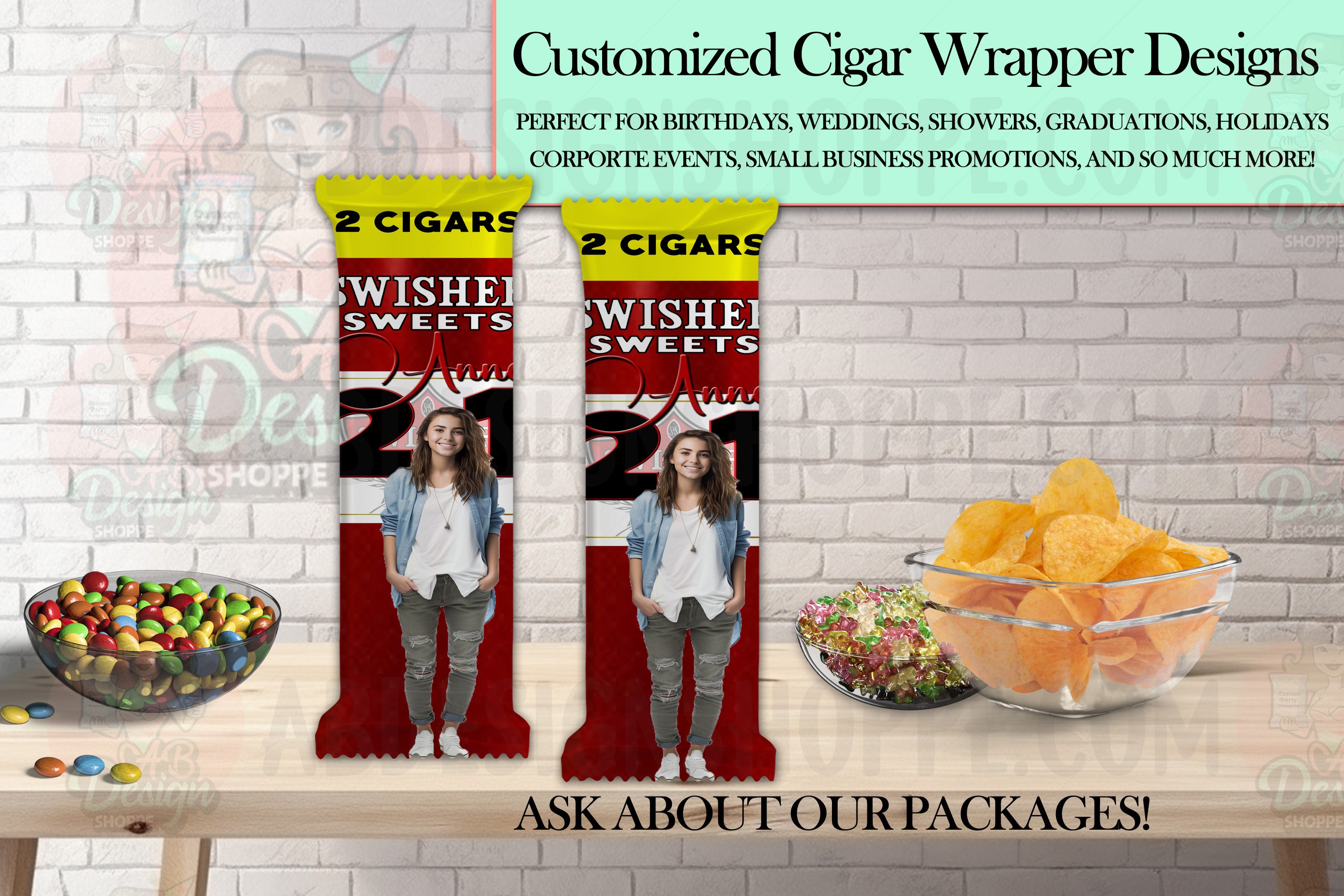This image is a close-up of a promotional advertisement set against a whitewashed brick wall, featuring a light-colored wooden trestle table. The focus is on customized cigar wrapper designs, highlighted in a light green block of text that reads: "Customized cigar wrapper designs perfect for birthdays, weddings, showers, graduations, holidays, corporate events, small business promotions, and so much more."

On the left side of the table, there is a colorful bowl of M&Ms featuring red, orange, yellow, and blue candies. Next to it, more towards the center of the table, there are two packages of Swisher Sweets cigars. These red-wrapped cigars have a bold yellow block text at the top that reads "Two Cigars" and include the image of a girl with shoulder-length brown hair, wearing a blue shirt over a white blouse, gray pants, and white shoes.

To the right, there are additional snack items including a bowl of orange chips and a small bowl of gummy bears in various colors: white, yellow, red, pink, and green. The bottom of the image features a caption that says, "Ask about our packaging." The entire scene is likely a computer-generated or skillfully assembled marketing image designed to showcase the product in a vibrant and appealing setting.